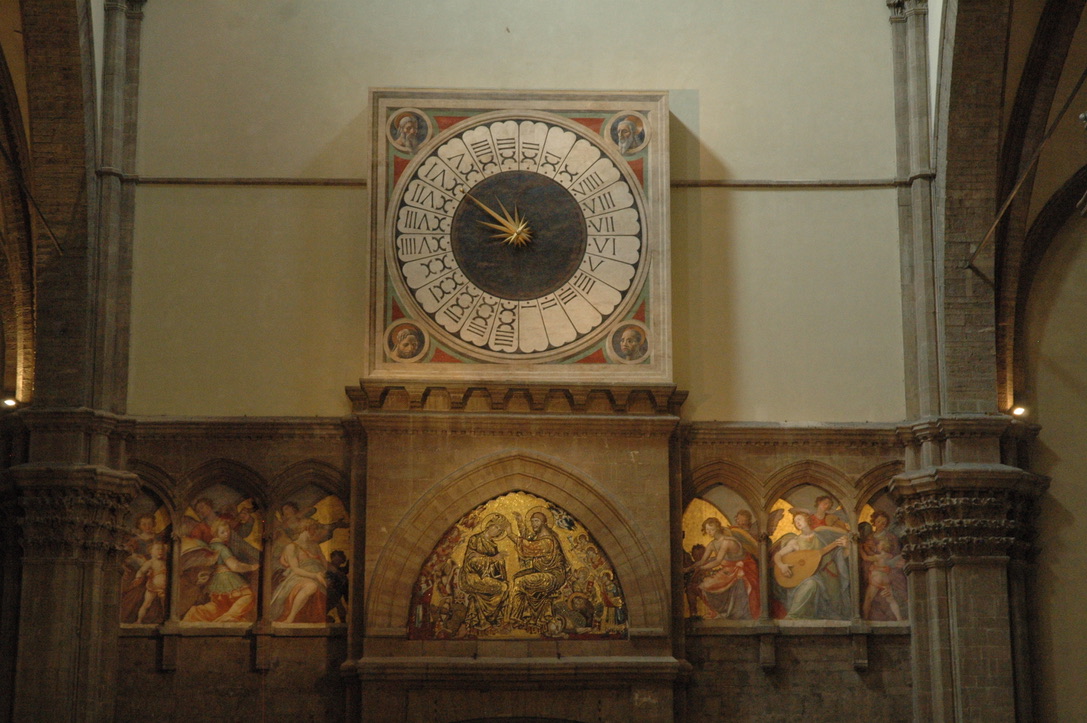The image depicts an interior scene from a historic church or ornately decorated vintage building, possibly from Europe, such as in Spain or Italy, reminiscent of 16th to 18th-century architecture. The focal point is a vintage Victorian-style clock set against a brown wall framed by two large, curved brown columns, each with a light fixture on the outer side. The clock itself features a light brown square frame adorned with four indistinct drawings in each corner and a brown border enclosing a white face decorated with leaf-like patterns and Roman numerals. At the center of the clock is a black area with a single elaborate golden hand. Below the clock, there are three small windows with religious depictions of children and angels. The wall beneath also includes tapestries or frescoes with religious imagery, including a central fresco showing a seated figure, possibly a depiction of Jesus or a Pope, blessing another seated figure, potentially Mary. The architecture includes frescoes with angels playing musical instruments, arches, and other elements typical of grand, historical churches visited in Europe. The detailed religious symbology and the antiquity of the decorations highlight the sacred and historic nature of the space.